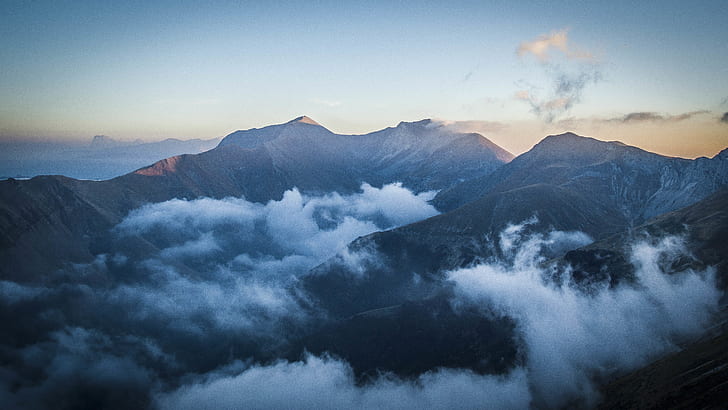This photograph captures an expansive aerial view of a rugged mountain range bathed in the fading light of sunset. The jagged, dark gray peaks of the mountains are interspersed with wispy white clouds, creating a dramatic contrast against the serene backdrop. The sky transitions from an aqua to light blue, and on the right side, it is lit with a warm pink and orange glow, hinting at the setting sun. Some mountain peaks reflect faint pink hues, indicating the last rays of sunlight. To the left, parts of the mountain range catch the sun's illumination, adding depth and dimension. In the hazy distance, another set of mountain peaks can be seen, blurred by the altitude. The overall scene suggests it was taken from a high vantage point, possibly from a helicopter, capturing the ethereal beauty of the mountains kissed by the evening light.